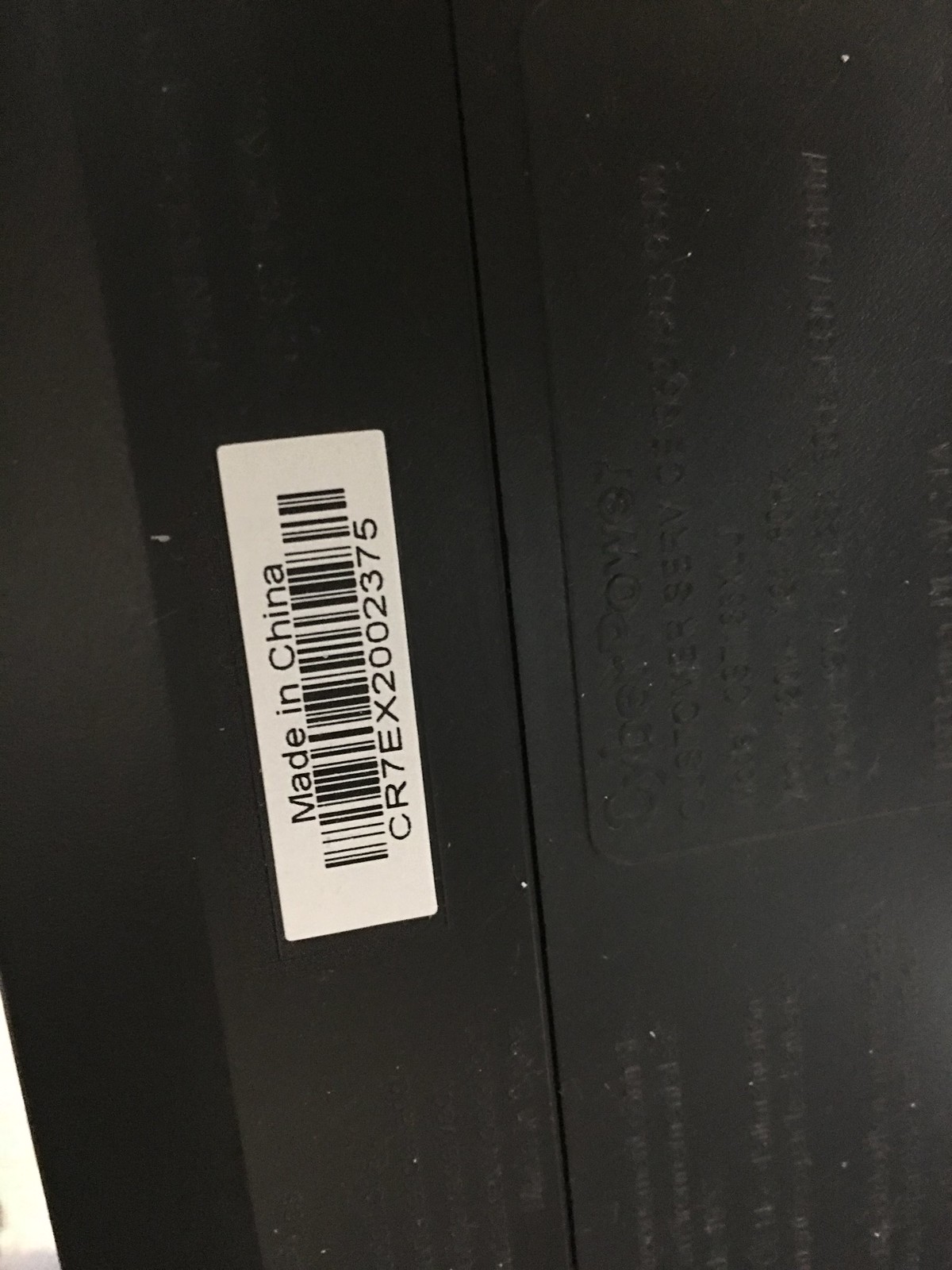This photograph is a close-up of the bottom or back of a black electronic device, possibly a laptop. The device is encased in a plastic housing and features a prominent white rectangular label. This label contains a black barcode with the accompanying serial number "CR7EX2002375" printed below it. Above the barcode, the label reads "Made in China." The image appears to have been taken at a slight angle, possibly a quarter turn counter-clockwise from its usual orientation. Additionally, there is embossed text on the plastic housing that includes phrases like "cyber power" and "service," although some of this text is not entirely legible. A vertical seam is also visible on the surface of the device.